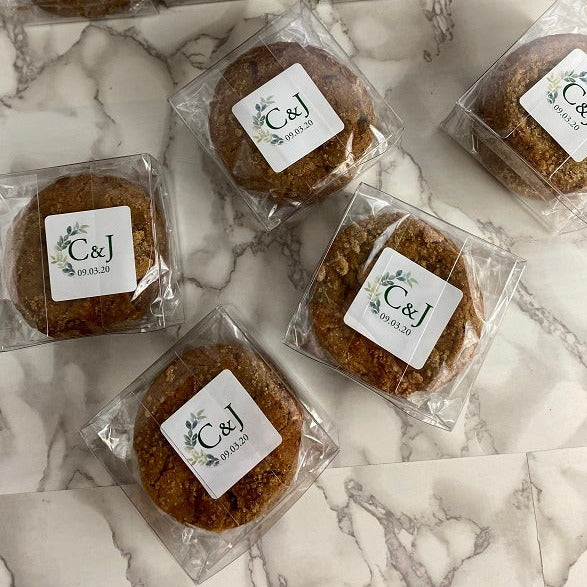The image features a close-up of several cellophane-wrapped pastries, possibly large cookies, arranged atop an intricate white marble table with prominent black veining and subtle splashes of beige, giving it a granite-like appearance. There are five visible pastries, but additional ones are slightly obscured at the top of the frame. Each pastry is encased in a rectangular plastic container, wrapped in clear cellophane, and bears a neatly positioned white square label. These labels prominently display the initials "C & J" in dark blue or black, with the date "09.03.20" beneath them, indicating they might be wedding favors. Decorative elements adorn the labels, with a delicate arrangement of green and yellow flowers and leaves arching upwards on the left side, adding a touch of elegance and personalization to the presentation.